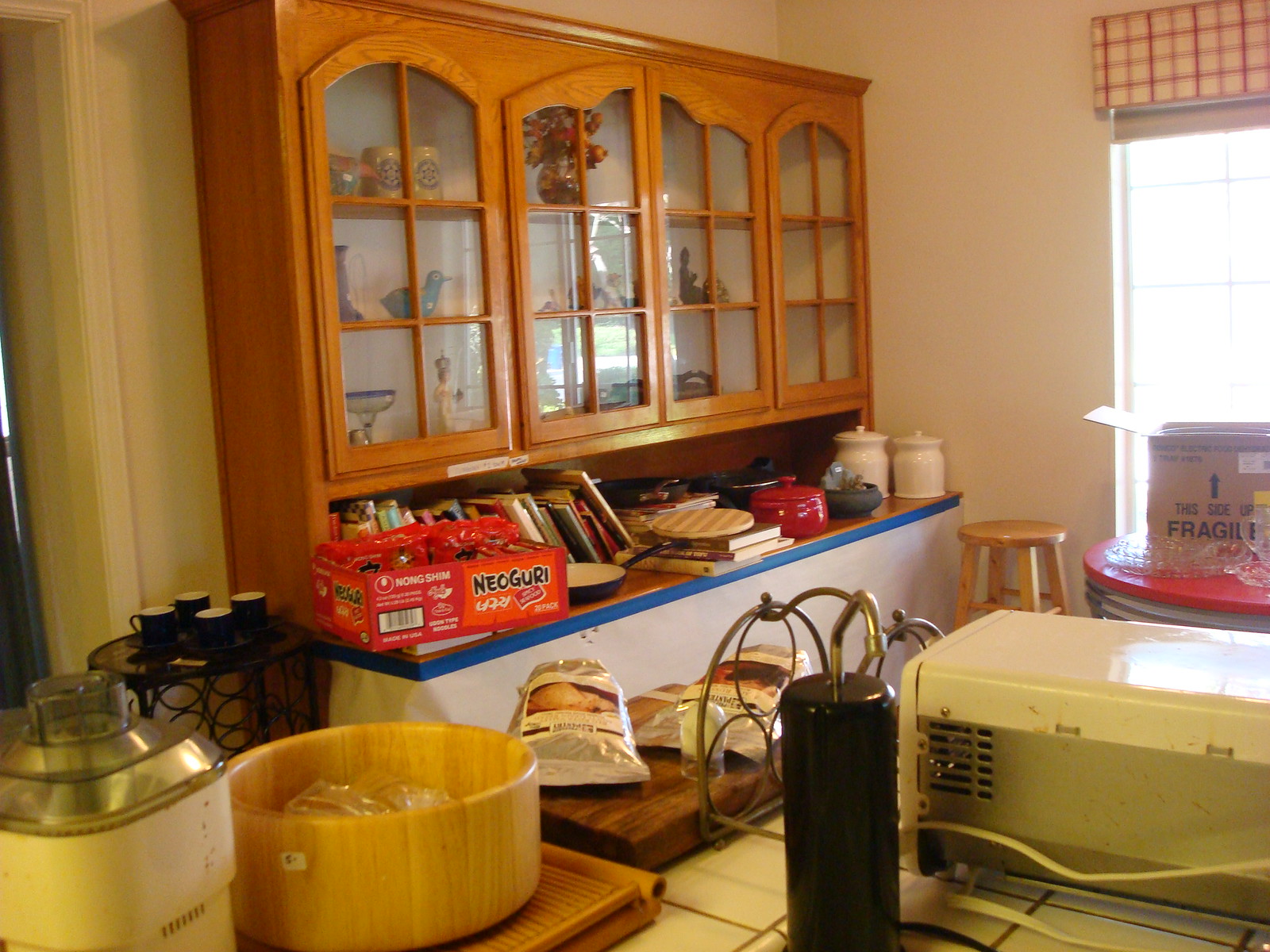The photograph captures a cozy kitchen scene. Prominently featured is a cabinet with upper glass-front doors showcasing decorative items including a vase of flowers, a glass bird, and a small statuette. Below the glass cabinets is a long wooden shelf lined with an assortment of recipe books, and at the far end of the shelf, two charming cookie jars add a touch of nostalgia. To the left side of the shelf sits a box of Neoguri noodles. 

In the foreground, a counter is partially visible. On it rests the back of a toaster oven, and beside it, a cutting board holding a couple of white packages. A deep wooden bowl containing unidentifiable plastic items adds a rustic touch to the scene. 

Across the room, beneath a sunlit window, stands a striking red Formica table, atop of which lies a cardboard box. The table's placement and color offer a cheerful contrast to the overall ambiance of this warm and inviting kitchen.